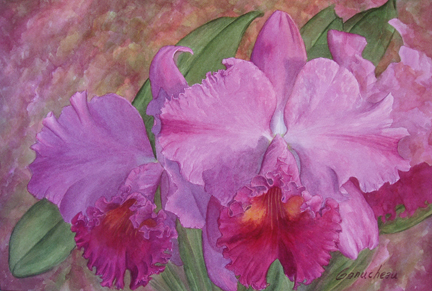The image features a detailed and expressive watercolor painting of flowers. The focal flower displays light purple petals with a richer, pinkish fuchsia center accented by touches of orange. Surrounding the flower are green, oval-shaped leaves that complement the main bloom. The background is an abstract blend of purplish-pink, tans, and browns, creating a harmonious and textured backdrop without any hyper-realistic elements. Brown accents further enrich the composition. A black, small signature in the lower right-hand corner reads "Gonucheau," suggesting the artist's name and adding a touch of sophistication. The artwork, which balances skillful detail and painterly abstraction, could easily find its place in an art gallery.